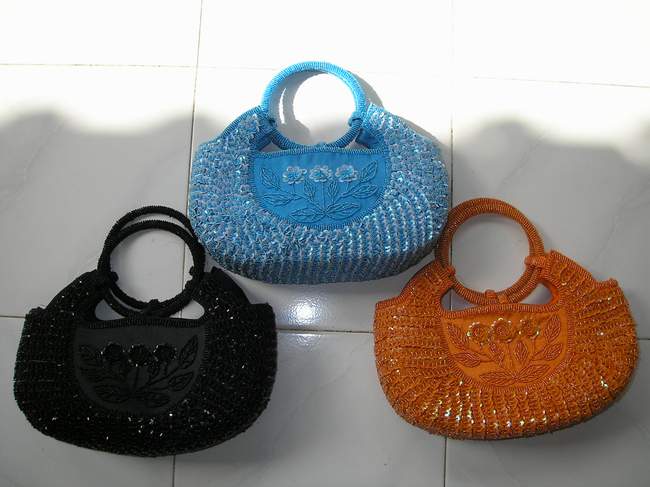This image captures three half-circle shaped handbags positioned on a white tile floor with faint gray veining or marbling. A light source behind the camera casts a shadow over the bottom three-quarters of the image. The blue handbag, centered at the top, features embroidered and sequined flower designs that lend a sparkly and reflective quality to its surface. Flanking it, the black handbag on the left and the brownish-orange, or perhaps reddish handbag, to the right also display similar floral embellishments. All three bags, woven to resemble straw, are decorated with intricate beaded flowers and sequins that catch the light. Each bag is equipped with two circular handles for carrying. The consistency in design across the bags—differing only in color—suggests a coordinated set, enhancing their visual unity.